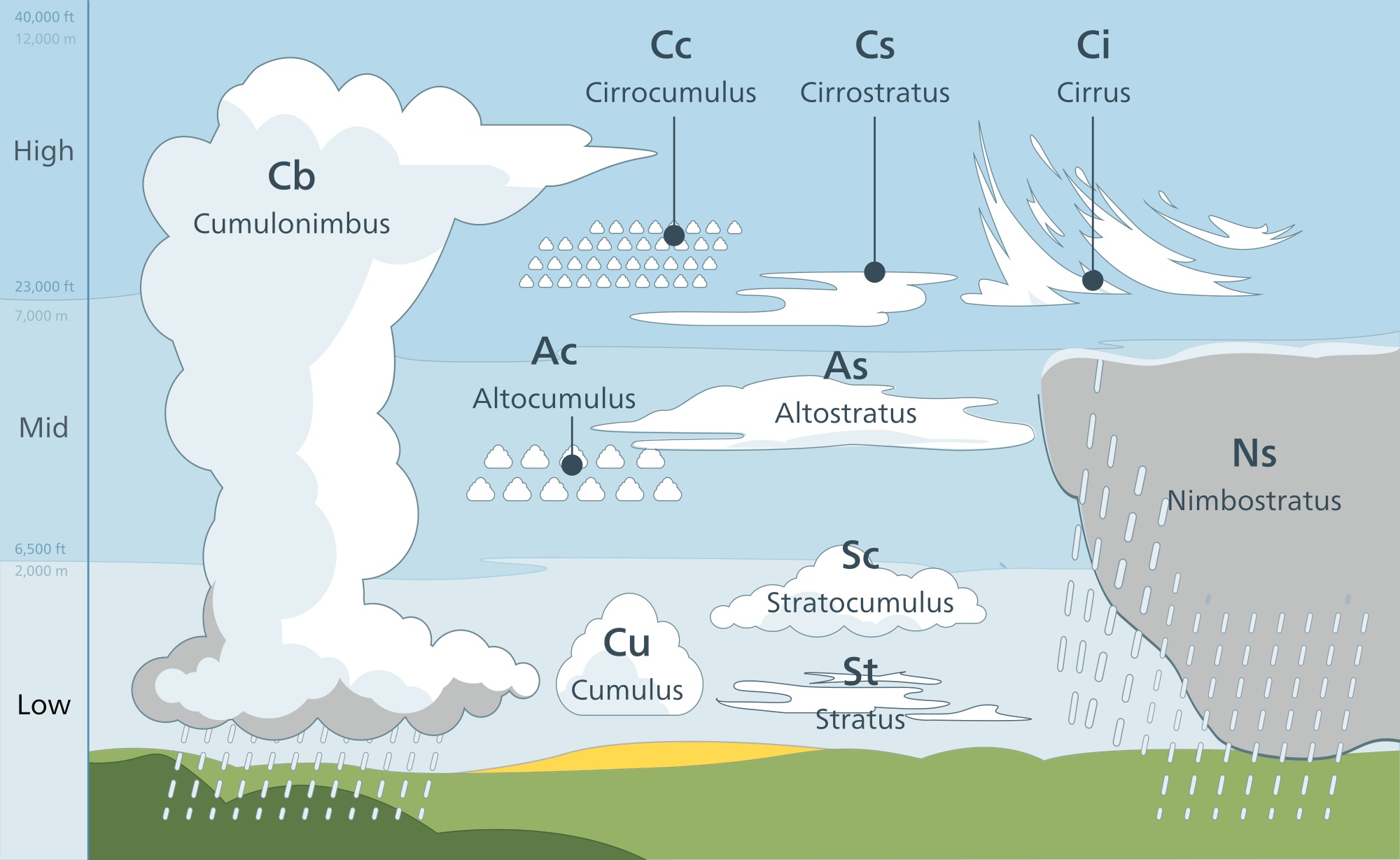This detailed textbook illustration provides a comprehensive overview of different cloud types, arranged in a horizontal rectangular frame against a predominantly blue background. The bottom portion features a thin strip of green grass representing the Earth's surface. The background transitions through three horizontal bands of blue, indicating the varying levels of the atmosphere: a dark blue upper third, a light blue middle third, and an even lighter blue bottom third.

On the left side of the image, a legend annotated in both feet and meters indicates the altitudes at which different types of clouds can be found. The legend is divided into three sections: "low," stretching up to 2,000 meters (6,500 feet); "mid," extending up to 7,000 meters (23,000 feet); and "high," reaching up to 12,000 meters (40,000 feet).

The clouds are illustrated from left to right within this framework. The most dominant feature is a towering cumulonimbus cloud (CB), spanning all three atmospheric levels and depicted with raindrops falling from its base. Nearby, a gray nimbostratus cloud (NS) occupies the lower and middle levels, also shown with raindrops cascading from it. Smaller clouds are distributed across different layers: cumulus (CU) near the bottom, altocumulus (AC) and altostratus (AS) in the middle, and cirrocumulus (CC), cirrostratus (CS), and cirrus (CI) at higher altitudes. Each cloud type is labeled with its name and abbreviation, providing a clear visual representation of their respective shapes and positions within the atmosphere.